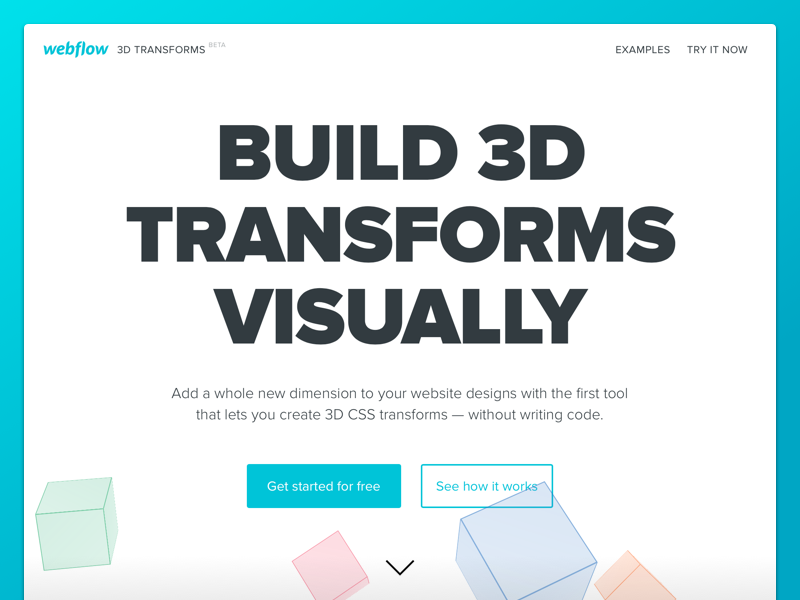This is a screenshot from the Webflow website, framed by a bold turquoise border. The central portion of the screenshot features a predominantly white background. In the upper left corner, the Webflow logo is displayed in italic turquoise font, which matches the border. Adjacent to the logo, the text "3D Transforms" appears in black, accompanied by a "beta" icon to indicate its experimental status. On the opposite end, the top right corner hosts navigation options labeled "Examples" and "Try It Now."

Dominating the center of the white section, in bold black typography, is the prominent headline: "Build 3D Transforms Visually." Below this, in smaller light gray font, a description reads: "Add a whole new dimension to your website designs with the first tool that lets you create 3D CSS transforms — without writing code."

Toward the bottom, two call-to-action buttons invite user interaction. The first button, filled in turquoise with white text, prompts users to "Get Started for Free." The second button, outlined in turquoise with turquoise text, encourages users to "See How It Works."